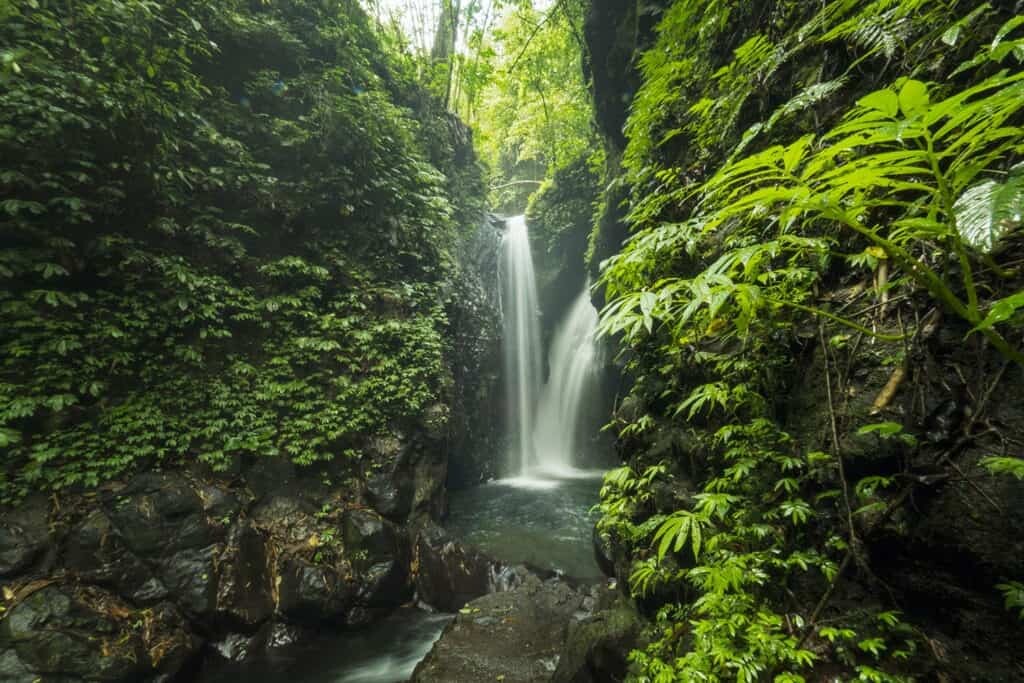This breathtaking photo captures a verdant waterfall cascading down a dramatic rocky landscape. The scene unfolds in a lush, green valley framed by two dark, rocky cliffs adorned with thick ivy and leafy vines. On the left side, the cliff is densely covered in ivy that flows down to about a yard above the rocky base. The right cliff shares a similar lushness, although some of the view is obscured by an abundance of leaves and smaller plants in the foreground. 

Centrally, the waterfall splits around rocks, creating a mesmerizing display of water plunging approximately 30 to 40 feet. The falls converge in a bubbling pool before continuing as a clear, green-hued stream that meanders through the valley floor. Sunlight filters through the canopy of bright green trees, casting a dappled light that enhances the serene atmosphere. The rocks around the waterfall, wet and gleaming, range in color from gray to black, contributing to the dramatic contrast between the dark stone and vibrant greenery. The background reveals further pockets of foliage and tall, light-colored trees, intensifying the tropical or East Asian exoticism of this picturesque, mid-afternoon scene.